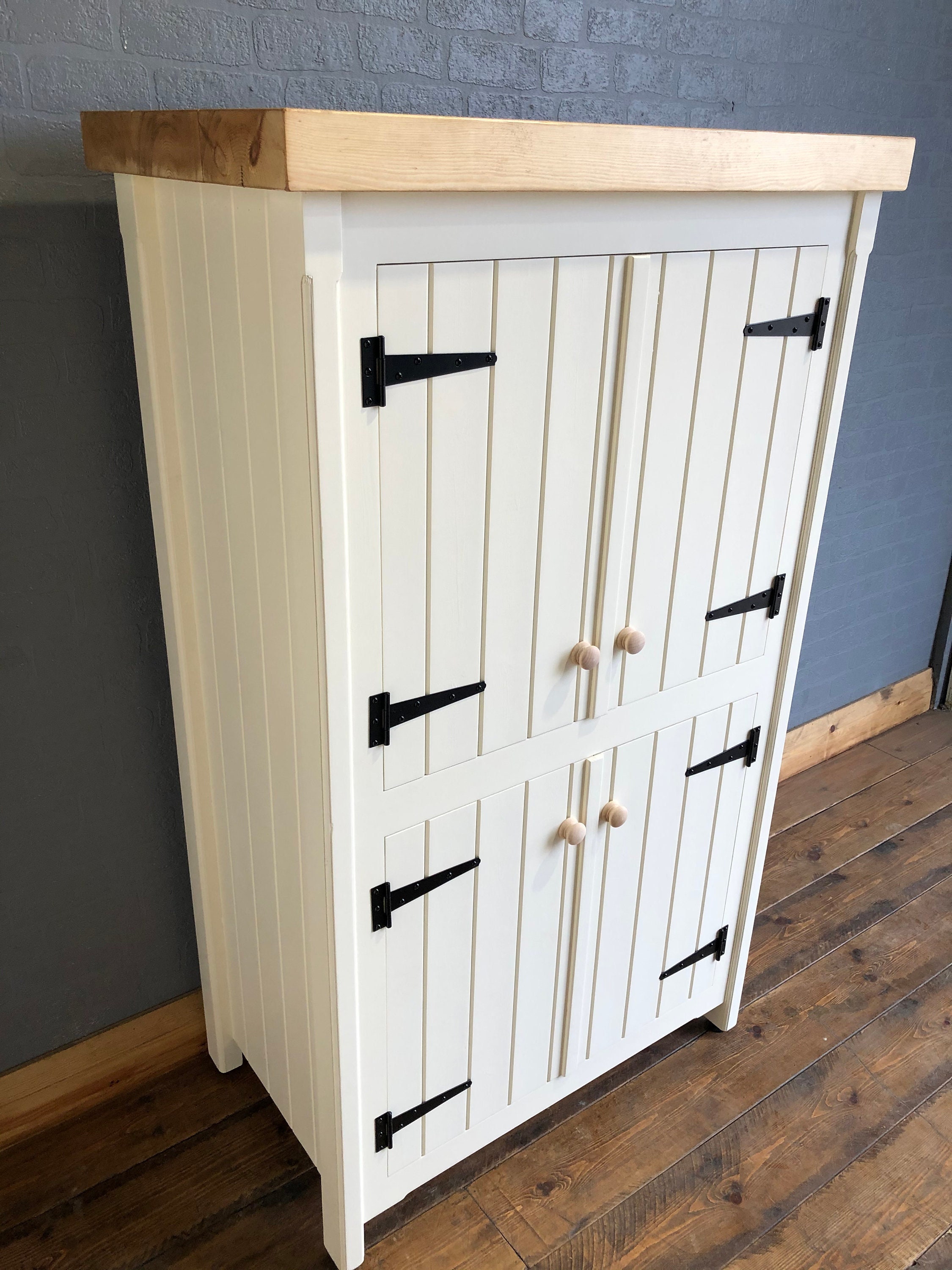The photograph captures an inviting corner of a rustic space with a warm wood floor and a blue painted brick wall, complemented by a lighter wood-colored baseboard at the base. The focal point is a tall, white French-style cupboard featuring a light wood top. The cabinet, divided into an upper and lower section, has four doors, each adorned with vertical panel detailing. Black hardware, including sizable hinges that span approximately half the width of the cabinet doors, accents the piece, along with four light wood knobs for opening the doors. The mixture of materials and colors - the rustic wood, white paint, and blue brick wall - creates a harmonious and cozy atmosphere.